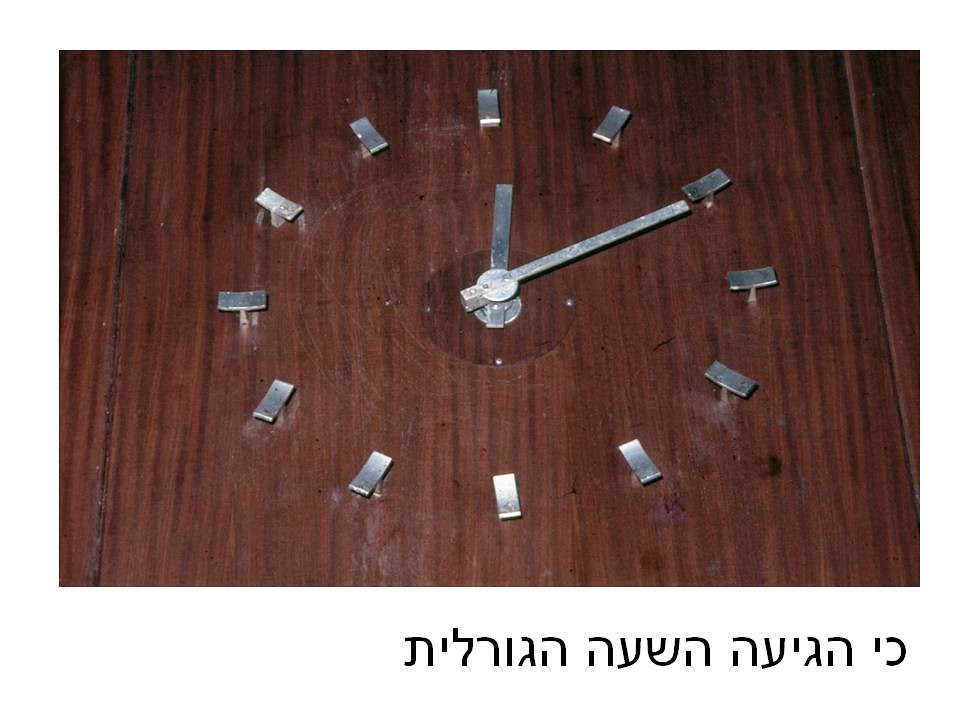The image showcases a vintage, wooden clock that appears heavily worn and in disrepair. This aged timepiece features 12 metal slits or markings in a circular arrangement to denote the hours, but many of these metal numbers are bent or misaligned. The clock's face is further marred by numerous scratches. The design is minimalist, featuring only a small, rectangular metal hour hand and a slightly longer, rectangular minute hand, with no second hand present. Below the clock, there is text written in a foreign language, inscribed in bold black letters. The overall condition reflects the clock's extensive wear and tear over time.